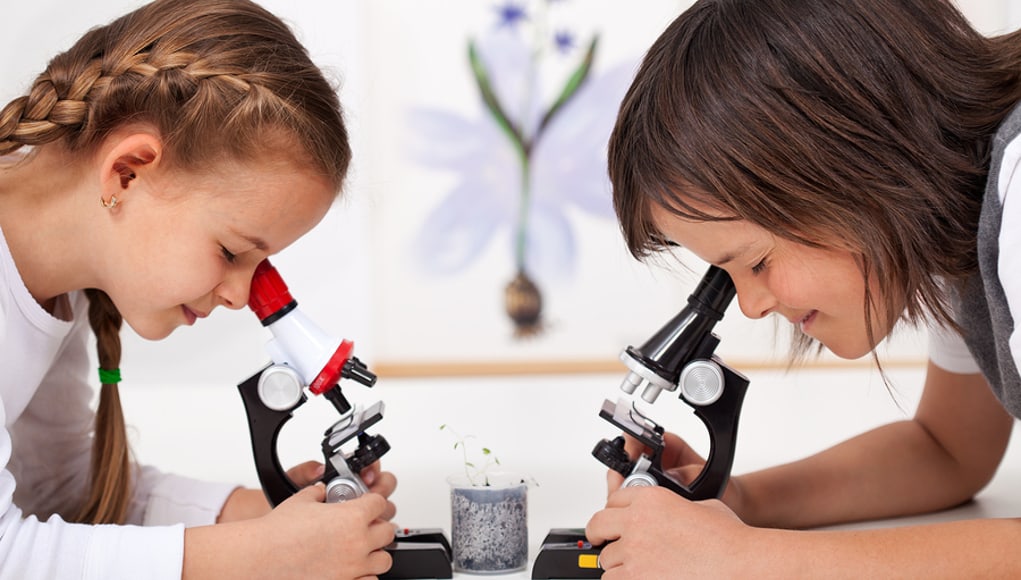This is a horizontal, rectangular color photograph depicting two young girls, likely in their early teens, deeply engaged in examining specimens through microscopes. They are positioned facing each other, each slightly in profile. The girl on the left, with reddish-brown hair styled in pigtails, is intently looking through a microscope featuring a red holder to the lens and a prominent white stripe. She is dressed in a long-sleeved white shirt and is grasping the lower part of the microscope, likely adjusting the focus. To her right, the other girl, with shoulder-length dark brown hair and bangs, wears a short-sleeved white shirt. She is similarly focused, peering through a black microscope with a notable white knob in the middle. Both microscopes have two lenses. Their concentration is evident as they manipulate the dials and possibly the slides to obtain better viewing angles. The background features a white wall adorned with a slightly out-of-focus poster displaying an emblem and a flowery symbol, adding to the academic ambiance of the scene. Both girls are smiling, reflecting their engagement and enjoyment in the scientific activity. The photographic style captures the realism and representational nature of the setting.